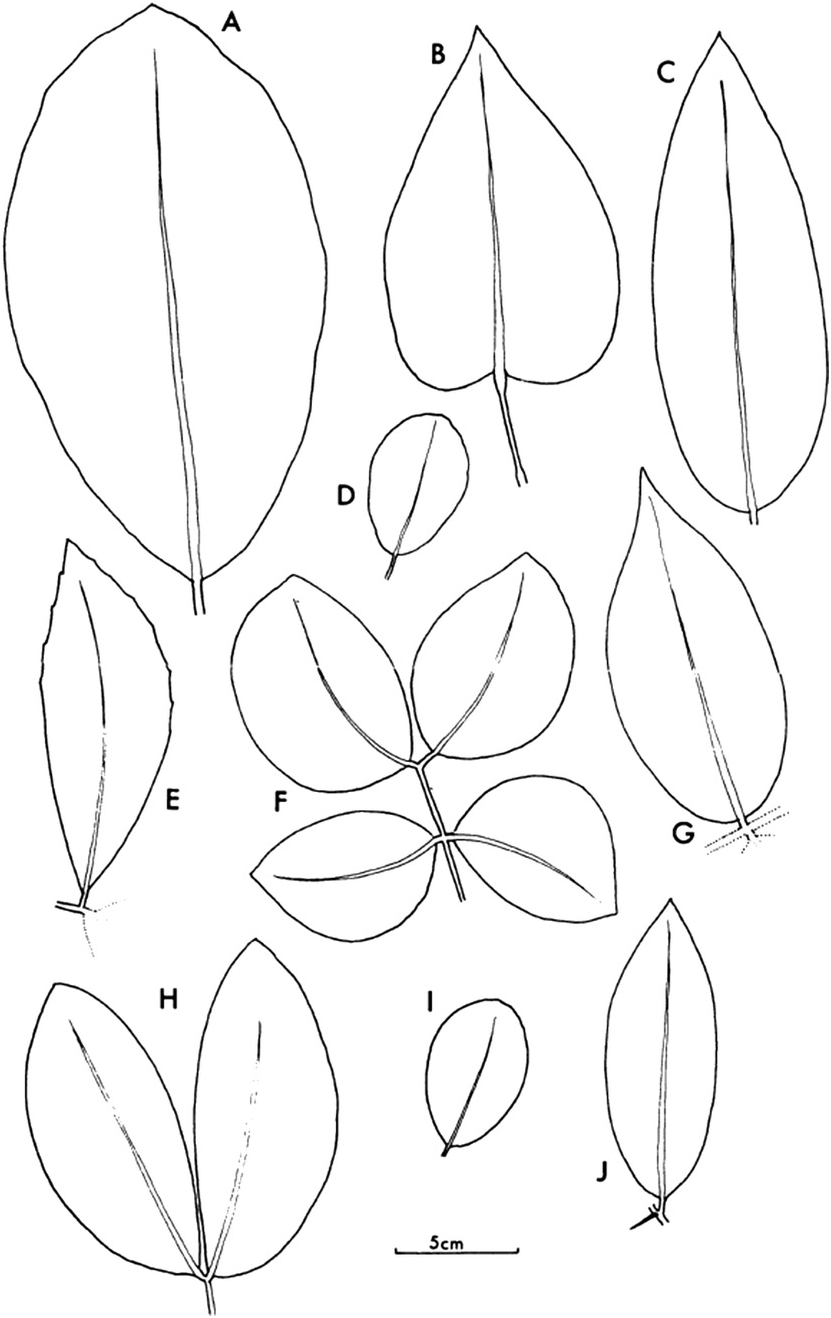This is a detailed black and white illustration depicting various types of leaves, each uniquely hand-drawn and labeled with letters from A to J. Every leaf is distinctly different in shape and size, showcasing a range from spade-shaped and oval leaves to a unique twig with four leaves sprouting out. Leaf E is particularly notable, with distinct jagged lines along its edge. The leaves are arranged in three rows: the first row contains four leaves labeled A, B, C, and D, with shapes varying from short and fat to heart-shaped and slender. The second row features three leaves, including one labeled F that consists of four smaller connected leaves positioned at the upper right, upper left, lower right, and lower left. The third row also has three leaves, including leaf H, which shows two connected leaves. For scale reference, the bottom of the image includes a 5-centimeter line. The illustration appears to be a chart, likely intended to identify different types of leaves based on their labeling.